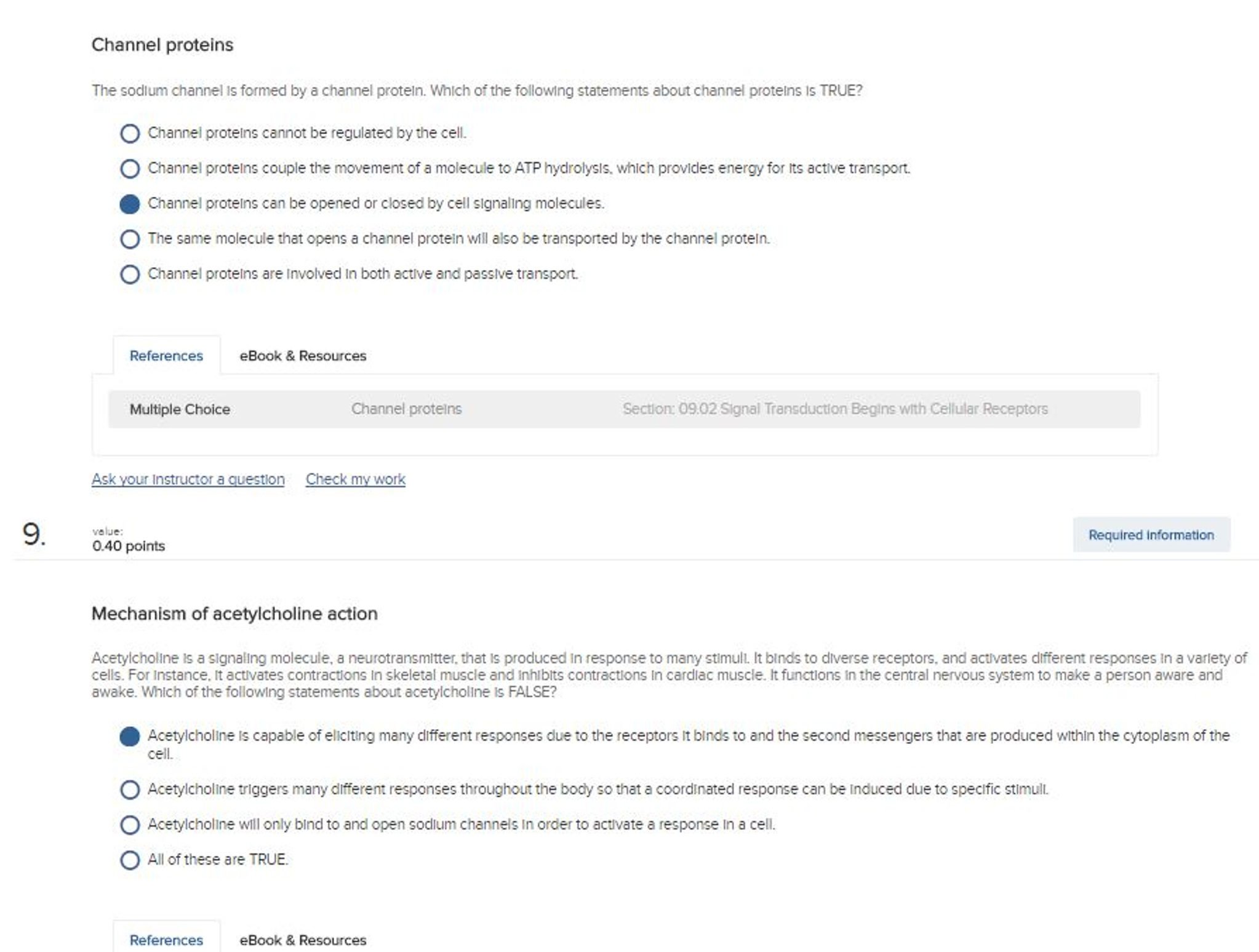**Detailed Caption:**

A detailed screen capture of an online test interface from what appears to be either a biology or chemistry course. The focus is on a multiple-choice question about channel proteins. The question reads: "The sodium channel is formed by a channel protein. Which of the following statements about channel proteins is TRUE?" Notably, the word "TRUE" is in all caps for emphasis. Five options are listed, each with a circular button for selection. The third option, "Channel proteins can be opened or closed by cell signaling molecules," is highlighted in solid blue, indicating it has been selected. The other options are:

1. Channel proteins cannot be regulated by the cell.
2. Channel proteins couple the movement of molecules to ATP hydrolysis, providing energy for active transport.
4. The same molecules that open the channel protein will also be transported by the channel protein.
5. Channel proteins are involved in both active and passive transport.

Below this, there is a reference section citing "E-books and Resources, multiple choice, channel proteins, section 09.02" which states "Signal transduction begins with cellular receptors." Additional links are provided for "Ask your instructor a question" and "Check my work."

Further down, the screen shows a question labeled "9," worth 0.4 points, titled "Mechanisms of Acetylcholine Action." The question text provides an in-depth description of acetylcholine as a neurotransmitter that binds to various receptors to elicit different responses, such as activating contractions in skeletal muscles while inhibiting them in cardiac muscle, and promoting alertness in the central nervous system. The question asks: "Which of the following statements about acetylcholine is FALSE?" The first option, indicating that acetylcholine can elicit multiple different responses via second messengers in the cytoplasm, is selected. There are two more unlisted options, with the last one stating "All of these are true" and remaining unselected. As with the previous question, there are references and e-book resources listed at the bottom.